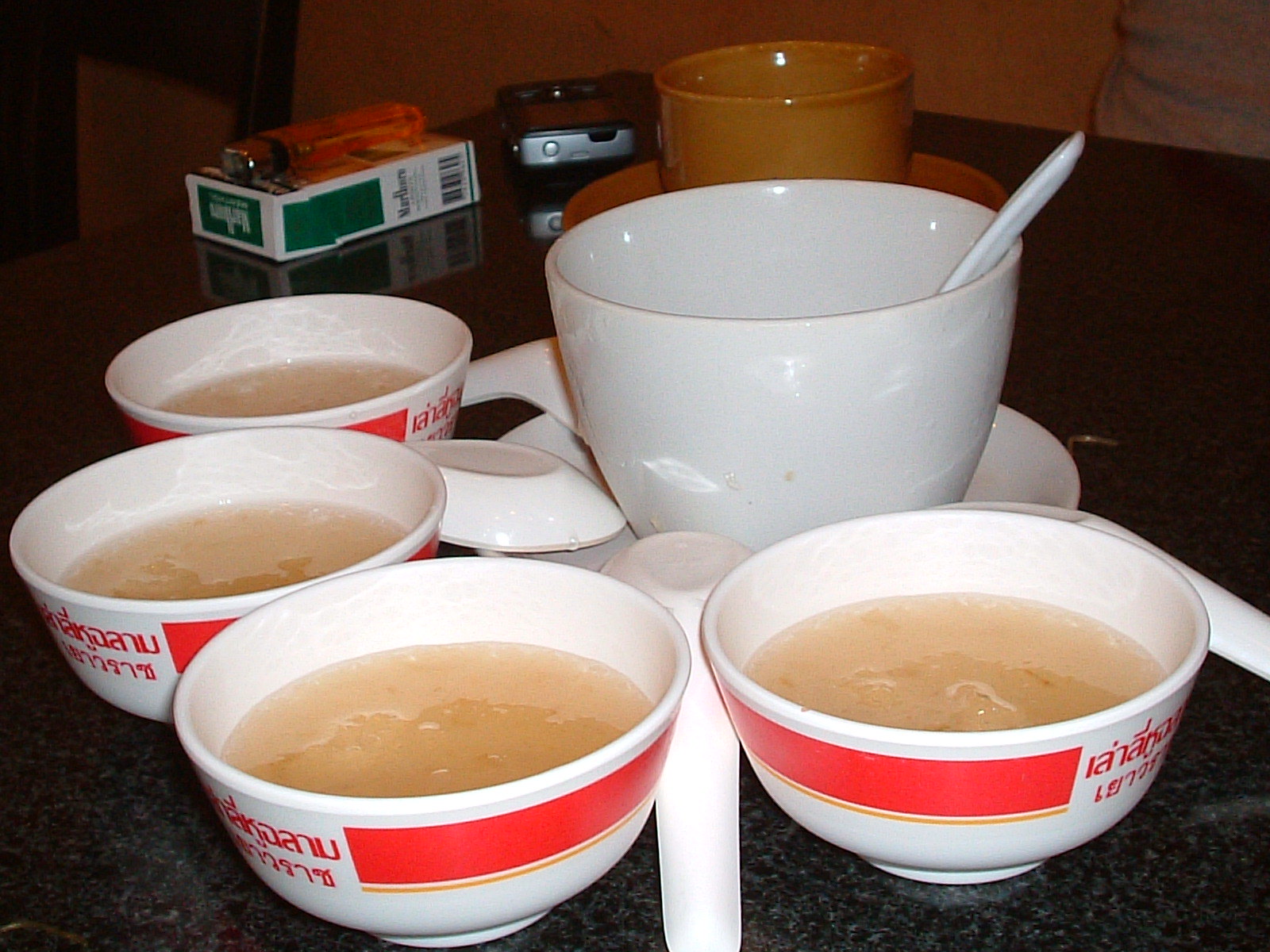This close-up image captures a table scene, prominently featuring a collection of bowls with soup. At the center, a large white bowl or mug rests on a white saucer, containing a creamy, milky peach-colored soup. A large spoon is stationed inside this central bowl, enhancing its noticeable presence. Surrounding the central bowl are four smaller white bowls, each adorned with red stripes and curvy, ornate characters likely from a Southeast Asian language such as Thai or Vietnamese. These smaller bowls contain a clear, brownish broth and are complemented by ceramic Asian-style soup spoons.

The backdrop of this image reveals additional items on a speckled dark brown or grayish table. Notably, a yellow or tan mug on a saucer stands behind the main bowl ensemble. To the side, there is a pack of Marlboro menthol cigarettes accompanied by a clear orange lighter placed on top. Additionally, an older digital camera or possibly a voice recorder is situated nearby, suggesting a snapshot from an earlier time, perhaps the early 2000s. This detailed scene indicates a meal setup, possible preparations for an Asian-style dining experience.